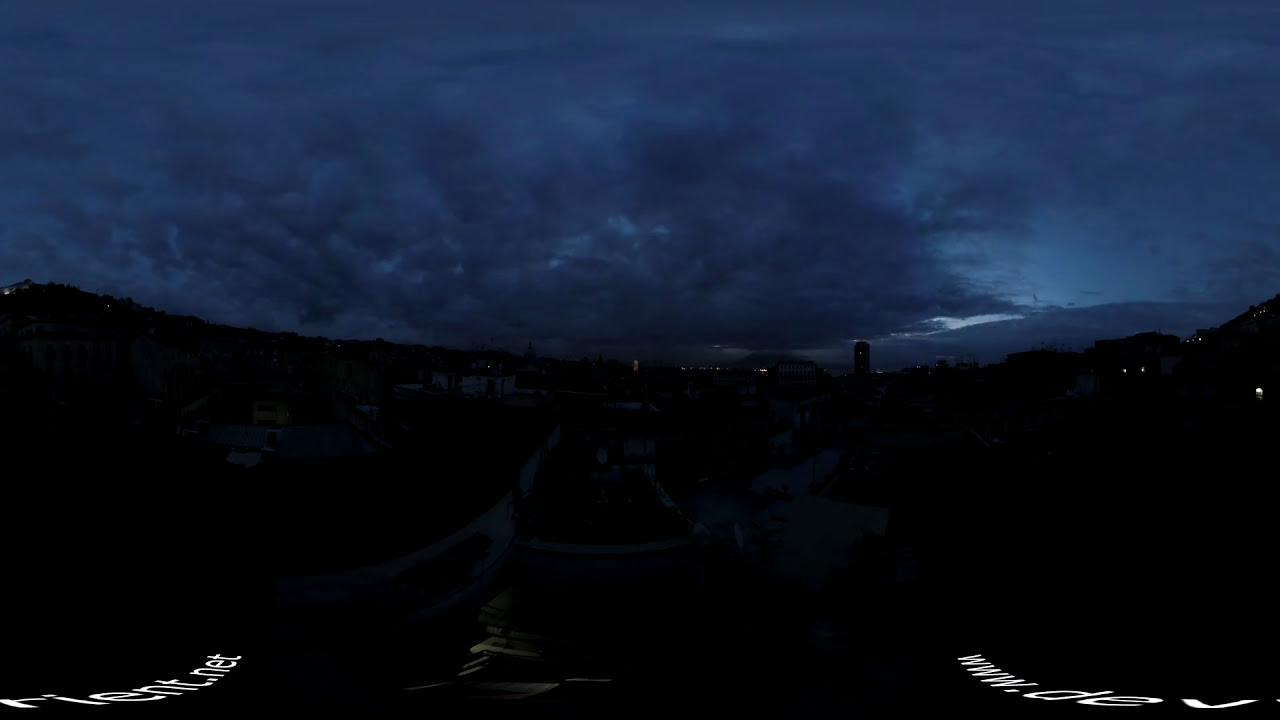The photograph captures an enigmatic cityscape at night, shrouded in darkness. The skyline is faintly visible against a dark blue, cloudy sky, with a subtle glow suggesting either a post-sunset or pre-sunrise atmosphere. Although most of the city appears as indistinguishable gray forms, a few small lights from windows punctuate the scene. Prominently, a tall tower-like structure rises on the right, juxtaposed with what seems to be an arched bridge in the distance. To the left of the tower, several spires peek upwards, adding to the intricate skyline. Both bottom corners of the image feature curved, illegible white text; on the left, it potentially reads "rient.net," while the right may bear "www.dev." These watermarks add an additional layer of intrigue to this dimly lit, almost mysterious urban tableau.